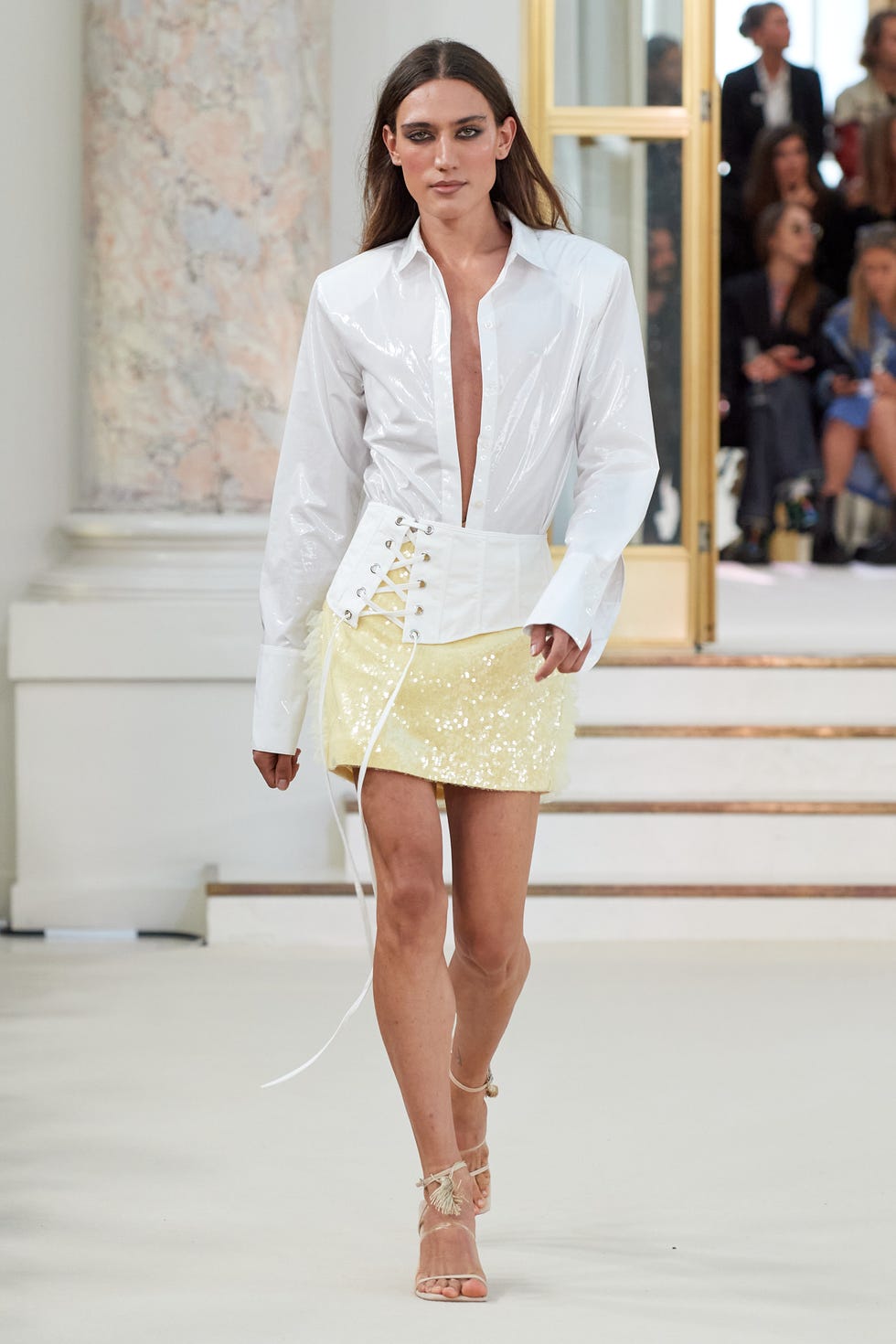In this color photograph, a young woman is modeling a striking outfit on a white runway, evocative of a fashion show or catwalk. The image, taken in portrait orientation, captures her full body from head to toe. She emanates a confident, focused demeanor with her serious expression and long, straight, dark brown hair cascading down her back. The model is walking towards the viewer, her hands hanging naturally by her sides.

She wears a shiny, long-sleeved, plastic-looking shirt that remains unbuttoned down the front, revealing a golden sparkly miniskirt beneath. The shirt's sleeves extend past her wrists and down to her fingers, adding an unusual and dramatic flair. This shirt is tucked into her short, yellow skirt, which is further secured by a bodice-like structure tied around her hips in an unconventional upside-down manner. Her footwear consists of strappy silver heels that elegantly wrap around her ankles.

To the right of the runway, there is a set of white stairs with wood-colored treads leading to a wood door at the top. Several people are seated on top of these stairs, perhaps either watching the show or involved with the fashion company, though they appear out of focus in the image. This photograph exemplifies a style of photographic realism, capturing the intricate details and the refined essence of fashion photography.